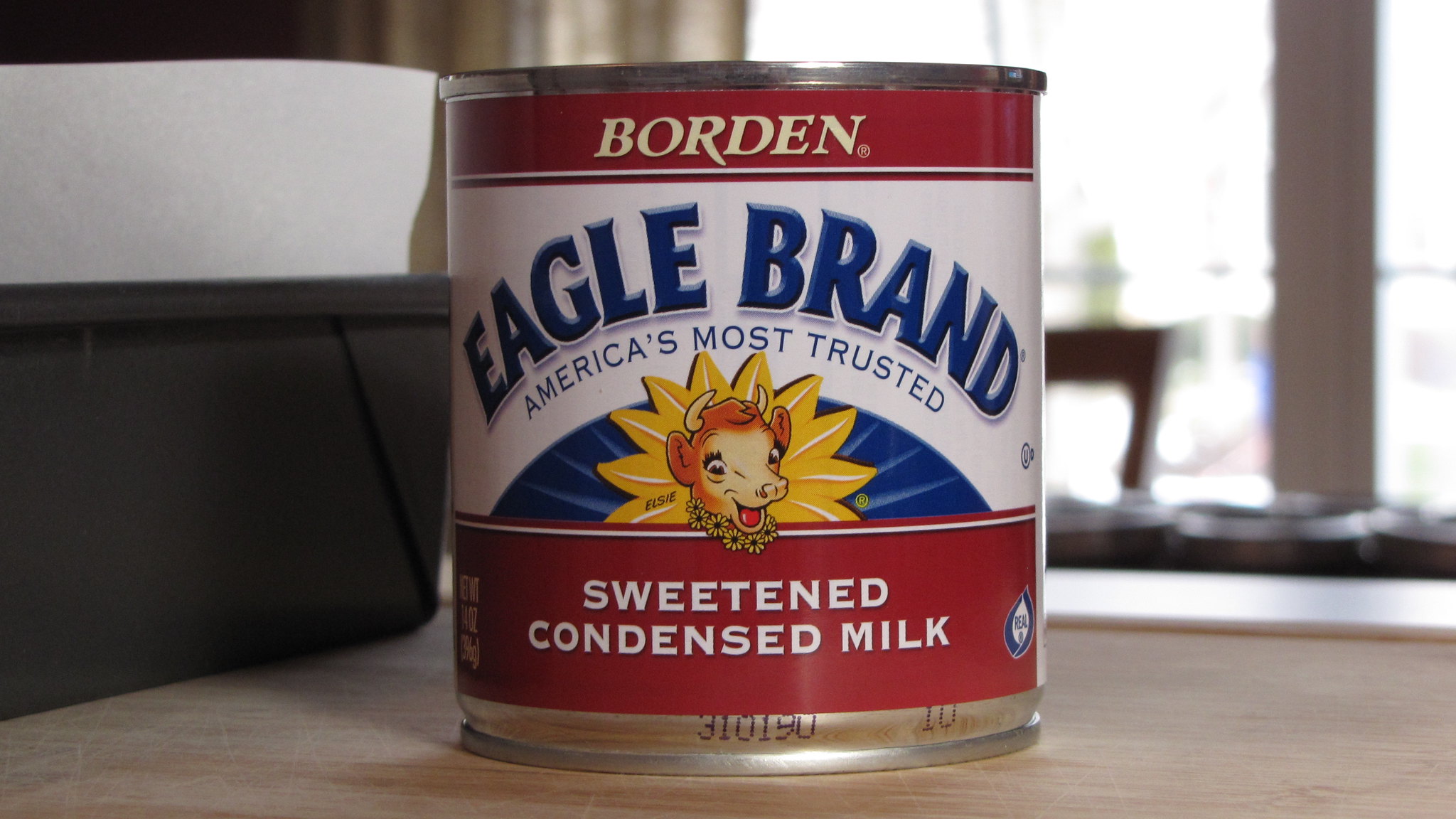The image depicts an up-close view of a can of Borden Eagle Brand Sweetened Condensed Milk, prominently positioned on a wooden table in a kitchen. The can features a distinctive label with several key elements: At the very top, a red stripe bears the words "Eagle Borden" in a serif font. Below this, the middle section is white with "Eagle Brand" displayed in bold blue letters, followed by the tagline "America's Most Trusted."

A central emblem showcases a sunflower with yellow petals, and at its heart is a detailed illustration of a brown cow with small horns, a light brown face, an open mouth showing its tongue, and a yellow flower garland around its neck. Below this, another red band with white text reads "Sweetened Condensed Milk." The can also includes the number "310190."

The setting is a kitchen, where the can rests on a wooden table. To the left of the can, a black plastic bucket containing a white object is visible. The background features a partially drawn brown curtain with an open window, allowing bright natural light to flood in, creating a light glare.